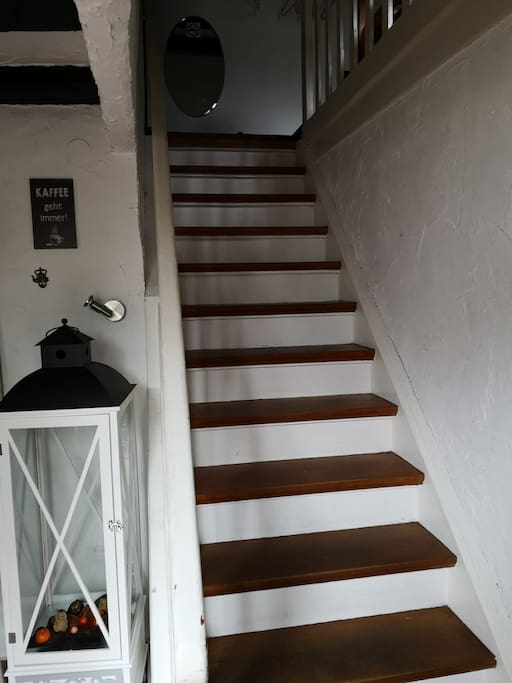This color photograph captures a wooden stairway positioned diagonally from the bottom right-hand corner, approximately at an 11:30 angle. The white risers and brown treads of the stairs contrast beautifully with the surrounding area. To the right of the stairway, there is a plain white wall, while on the left, a white railing is visible. Below this railing, the area extends towards a hallway with various details. The left side of the image reveals a tall, rectangular white cabinet with a glass exterior beneath each panel; inside, a variety of colored rocks—orange, red, white, and gray—can be seen. Above this cabinet, there are two metal fixtures: one resembling a faucet and the other a horn. A brown sign with white text reading “CAFE - K-A-F-F-E-E” hangs on the wall, alongside a picture of a steaming coffee cup. Farther back into the scene, there is a silver-handled door and, nearby, an oval mirror or picture hanging at the top of the stairway. Both the white and wooden bannisters on either side add an inviting contrast to the space.